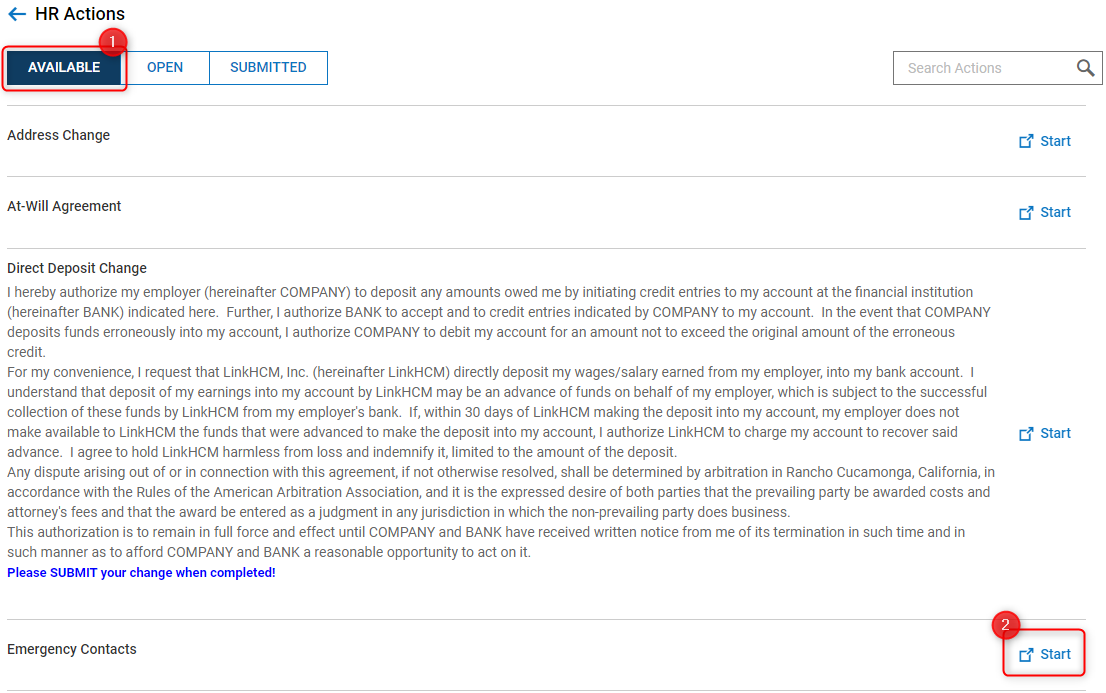The image depicts a user interface form with an "HR Actions" label on the top left next to a blue arrow pointing left. Below this header are three buttons: the first is blue with white text labeled "Available" and marked with a red circle containing the number "1". The second and third buttons are labeled "Open" and "Submitted" respectively. To the right of these buttons is a search bar labeled "Search Actions".

Underneath this section, a gray horizontal line separates it from the next line of content, which lists an "Address Change" action with a star icon on the right. Following this is another line labeled "At Will Agreement" with its own star icon situated far to the right. A subsequent gray line appears below these entries.

Further down, the form includes a section labeled "Direct Deposit Change," followed by detailed legal text. The text starts as: “I hereby authorize my employer, hereinafter company, to deposit any amounts owed me by initiating credit entries to my account at the financial institution, hereinafter bank, indicated here. Further, I authorize bank to accept and to credit entries indicated by company to my account. In the event that company deposits funds erroneously into my account, I authorize company to debit my account for an amount not to exceed the original amount of the erroneous credit." The legal text continues with more terms and conditions.